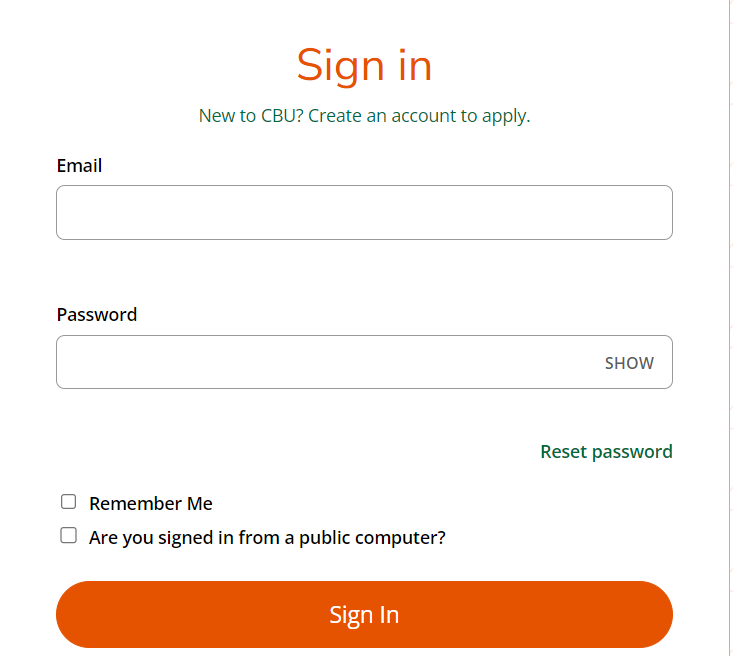This image shows a clean, white-background user interface for the CBU login and account creation page. On the right side of the image is an extremely thin black line. At the top center of the page, the text "Sign In" is prominently displayed in orange. Below this, in green, it reads, "New to CBU? Create an account to apply." 

The page then has a black-labeled "Email" input field with a thin black outline. Below the email field is a "Password" field, structured similarly with a thin black outline, and containing the capitalized gray text "SHOW" on the right side. 

To the right, in green text, is the "Reset Password" link. Below this, on the left side, are two stacked checkboxes. The top checkbox reads "Remember me," and the bottom one reads "Are you using a public computer?" Both checkboxes are currently unchecked.

At the bottom of the form is a large, orange "Sign In" button with white text. The color scheme of the interface consists mainly of white, orange, green, black, and gray. The overall design is minimalistic and focused on facilitating user login and account creation for CBU, although the function or nature of CBU itself is not further explained in the image.